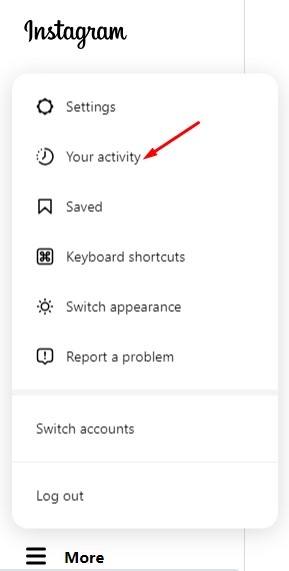This image is a partial screenshot of the Instagram desktop website displayed in light mode, featuring a prominent white background. At the top of the screenshot, the word "Instagram" is visible, written in a black cursive font. The screenshot focuses on a specific area, highlighting a white pop-up overlay that obscures part of the underlying content. This overlay appears to be a result of an interaction, such as a click, revealing several clickable options within the pop-up menu.

1. A gear icon labeled "Settings."
2. A clock icon labeled "Your Activity," accentuated by a red arrow pointing towards it, indicating it as the key focus of the image.
3. A bookmark icon labeled "Saved."
4. An X icon labeled "Keyboard Shortcuts."
5. A sun icon labeled "Switch Appearance."
6. An exclamation point icon labeled "Report a Problem."
7. Additional options at the bottom of the pop-up include "Switch Accounts" and "Log Out."

The detailed annotations and highlighting in the image suggest that the primary intent is to draw attention to the "Your Activity" option, as denoted by the red arrow.